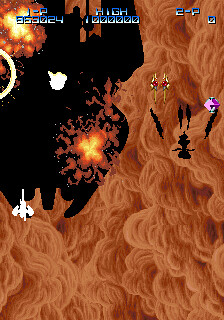In this detailed screenshot from a shoot 'em up video game, players find themselves amidst expansive sand dunes, showcasing an intense scene brimming with action. Dominating the background, a significant blaze engulfs a massive tar pit, sending fiery explosions cascading into the air. The game's high score currently stands at an impressive 1,000,000 points, with player 1 achieving a notable 853,024 points, while player 2 remains at a stark 0 points. Central to the chaos, two indistinct characters, one purple and one red, battle through the inferno, their forms barely discernible amidst the tumultuous surroundings.